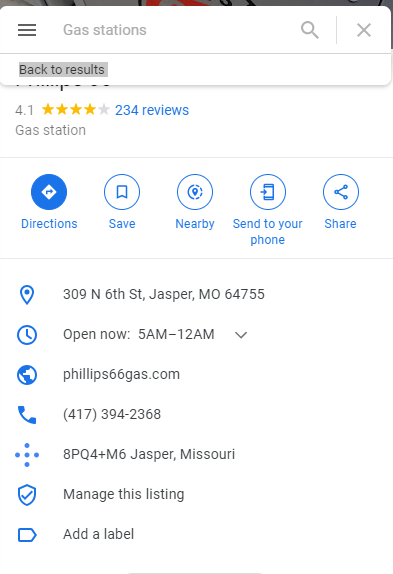This screenshot appears to be taken from a mobile device, likely a tablet or smartphone, given the compact layout. At the top, there are three horizontal black lines in a white rectangle, suggesting a menu icon. The title "Gas Stations" appears in gray, followed by a magnifying glass icon for search and an "X" next to a gray line.

Highlighted below this, a section reads "Back to results" with a gray background and black text. The first business in the list is partially obscured but shows a rating of 4.1 out of 5, with the stars colored gold. There are 234 reviews in hyperlinked blue text, and the category is listed in gray as "Gas station."

Below this, there are several interactive buttons: a dark blue circle with a white diamond containing a right-pointing blue arrow labeled "Directions," a white circle with a blue border and a bookmark symbol labeled "Save," and a pin icon with dashed lines labeled "Nearby." Additionally, there's a blue circle with a phone icon and an arrow labeled "Send to your phone," and another blue circle with a share icon consisting of three circles connected by lines.

Further down, the address is displayed: "309 N 66th Street, Jasper, MO 64755." An open hours indicator shows "Open now" with hours listed as "5 AM to 12 AM." A web link to "phillips66gas.com" is present along with a telephone number: "(417) 394-2368."

Additional elements include a diamond made of five spaced-out blue circles with the text "APQ 4+M 6" and "Jasper, Missouri." There's a shield icon with a check mark labeled "Manage this listing" and a right-pointing arrow labeled "Add a label."